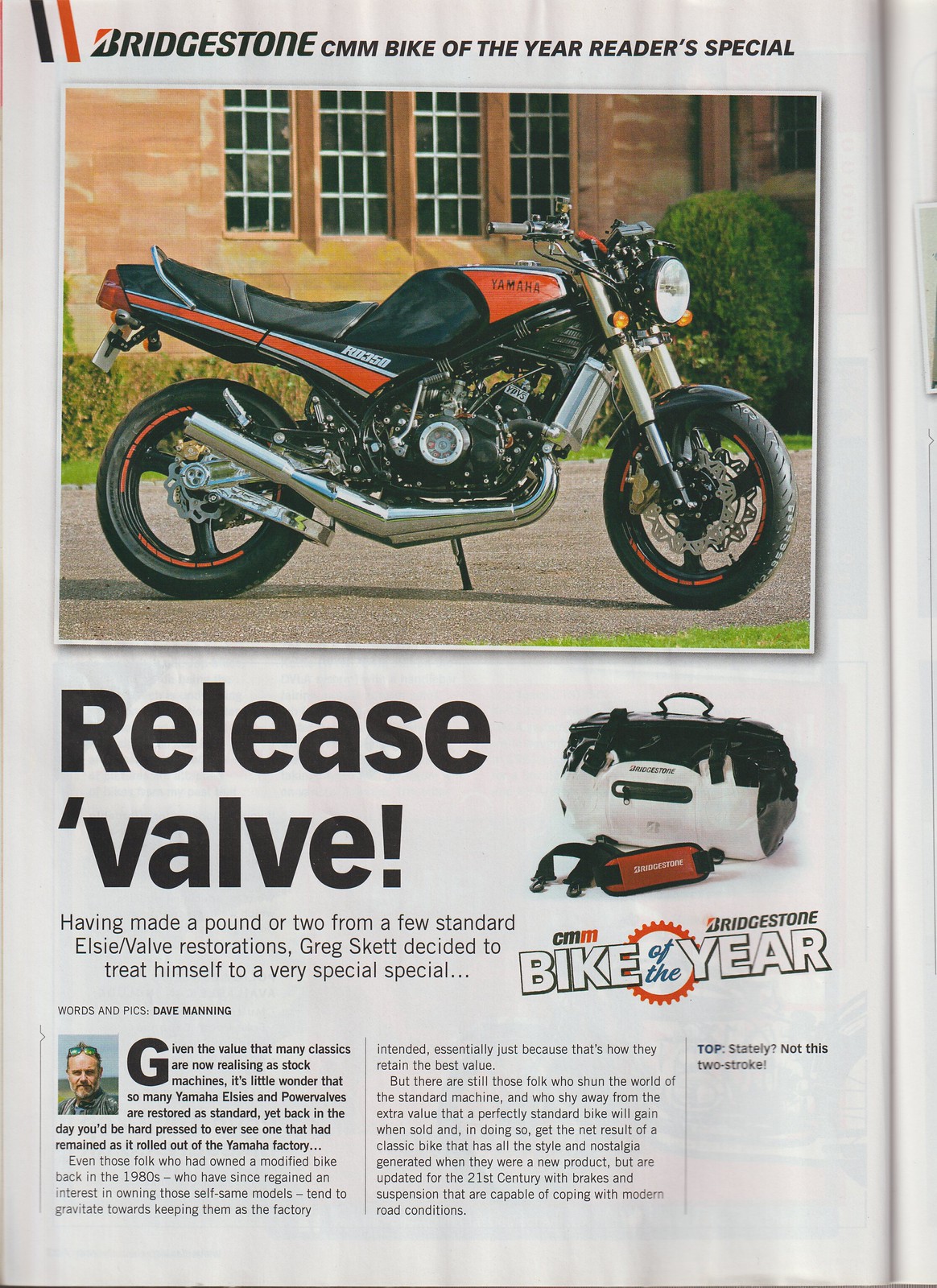This image is a detailed advertisement for a Yamaha motorcycle, prominently featured on a magazine's left-hand page. The model showcased is a vintage black and red Yamaha R0350, positioned upright on a kickstand on a gravel surface, bordered by a building and bushes in the background. The advertisement is topped with the title "Bridgestone CMM Bike of the Year Reader Special," emphasizing its prestige. Below the motorcycle image, the title "Release Valve" introduces an article highlighting Greg Skett's reward to himself for successful LC valve restorations. The text suggests a connection to Bridgestone equipment, featuring a branded duffel bag and possibly a belt. The article, credited to Dave Manning, offers an in-depth discussion and includes his picture.